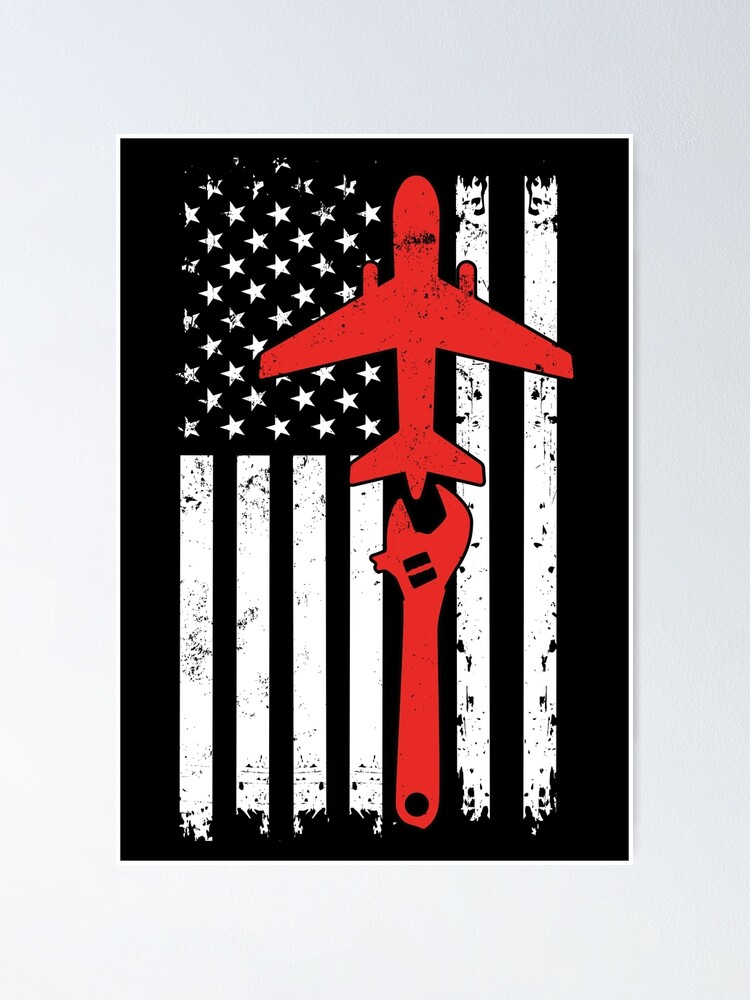The image depicts a black and white American flag with a distressed, vintage appearance, featuring frayed edges and faded stripes. The flag, adorned with 50 stars, hangs from the left side, with the stripes running vertically. Positioned against a white wall, the scene showcases a red passenger jet from a top-down perspective, revealing its two engines, fuselage, wings, and tail. Below the plane, a red crescent wrench appears aligned with the tail, as if prepared to fix the aircraft. The entire composition is rendered as faux-worn, suggesting a deliberate design choice to evoke a rough, aged aesthetic.